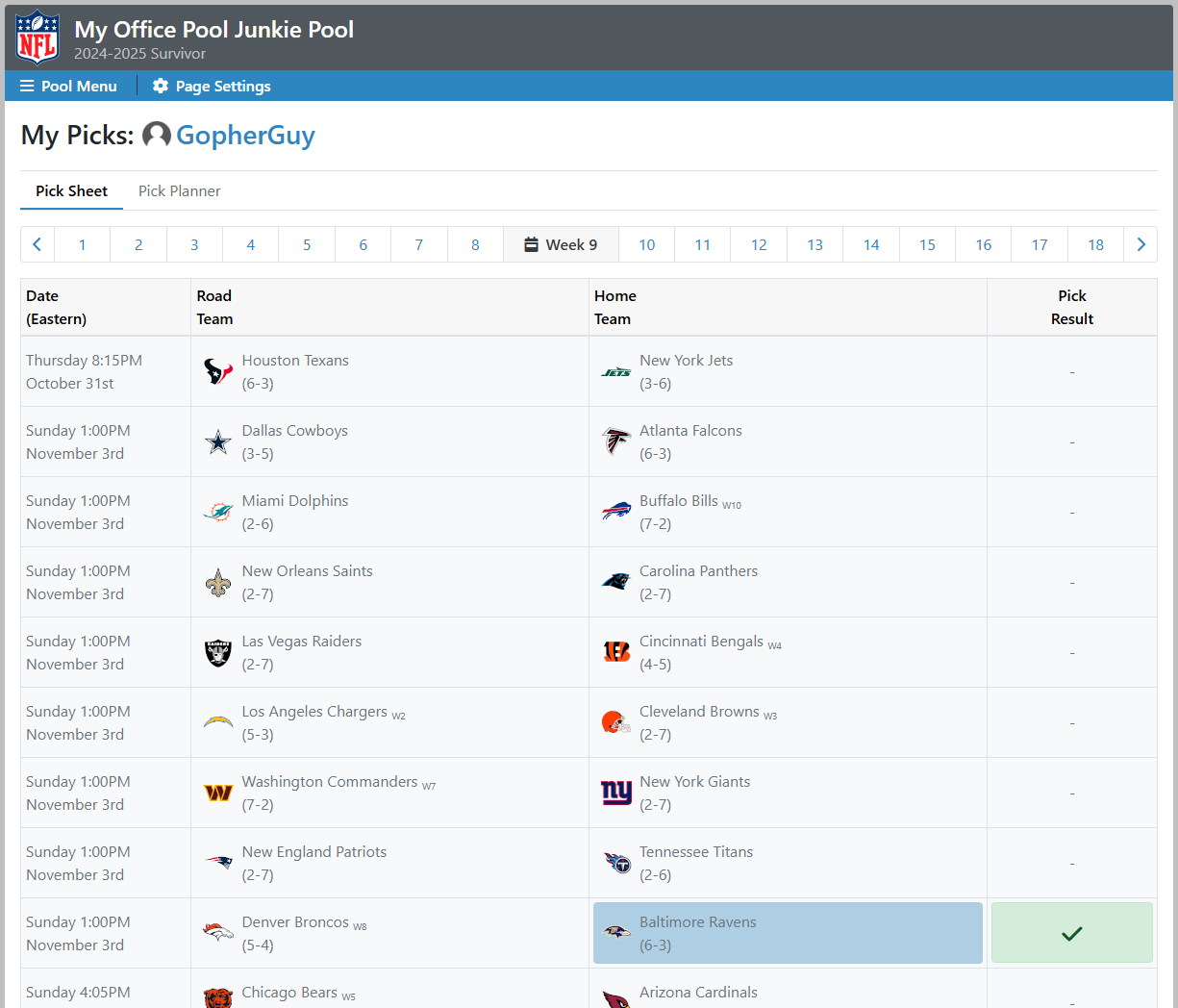The image displays a detailed schedule for a particular person's sports picks, titled "My Pics: Z Soaps" in the upper left-hand corner. There is a navigation button labeled "Week 12" in the upper section, flanked by arrows indicating navigation to previous and upcoming weeks. Below the navigation section, there are tabs. The "My Pics" tab, highlighted in black text, is active while the "Pic Planner" tab, written in blue, is inactive.

Within the "My Pics" section, the content is organized into four columns labeled Date, Eastern, Road Team, Home Team, and Pick Results, each enclosed in a white rectangular box. Under these categories, the schedule lists specific matchups. For instance, the game on the list includes the Chicago Bears (record 4-7), represented by their logo on the left, playing against the Detroit Lions (record 0-10-1), represented by their logo on the right. This format repeats for various games and dates.

Additionally, it is noted that the individual has marked the Dallas Cowboys game with an "X" in the pick result column, indicating a particular interest or selection for that matchup. The image effectively outlines the user's sports schedule preferences and picks for a specific week.